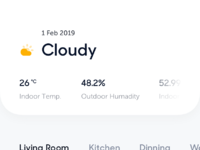This is a small, extremely blurry screenshot of a weather app, though it is unclear whether the app is on a phone, a computer, or another device due to the indistinct nature of the image. The screenshot appears to be clipped oddly, obscuring some critical information. 

Prominently featured is a yellow cloud icon, possibly with a sun behind it, suggesting partly cloudy weather. To the right of this icon, the date "1 February 2019" is visible, followed by the word "cloudy." Below this, there are several pieces of data: an indoor temperature reading of 26 degrees, an outdoor humidity of 48.2%, and another temperature reading of 52 degrees, though the context for this is cut off. 

Further down, there are option labels for different rooms: "living room," "kitchen," "dining," and a fourth option that starts with a "W," though the full word is not visible. The text is partially cut off at the bottom. The "living room" label is dark grey, possibly indicating it is the currently selected option, while the other room names are in light grey.

The overall image quality is extremely blurry, not grainy, which makes it difficult to ascertain finer details or the nature of the app.